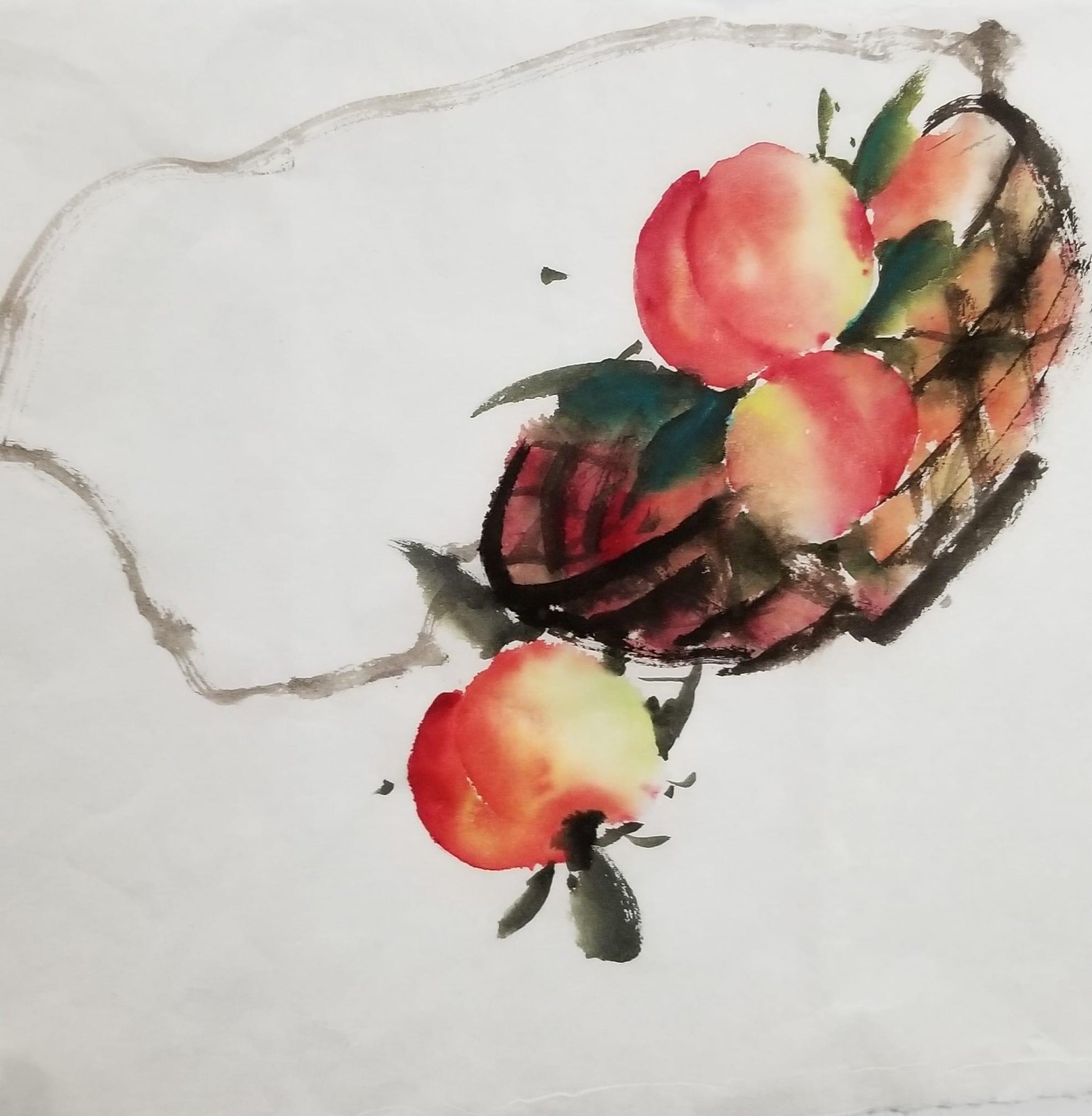This vibrant watercolor painting on slightly aged, white paper depicts a picturesque scene of peaches in and around a woven basket. Three prominent peaches, painted in shades of reddish-orange with yellow highlights, dominate the composition. Two peaches are nestled in the intricately detailed basket, which features black outlines suggesting a wire or woven structure. Green leaves and stems extend from the peaches, adding a touch of freshness to the artwork. The basket, resembling a small boat with its brown and red hues, appears to be tipping over, causing one peach to already tumble out, while the others seem poised to follow. Adjacent to the basket, a single peach, fully ripened with a blend of peach and yellow tones, rests beside it on the table, complete with a dark stem and lush green leaf. Connected to the basket is a delicate string, sketched with light black lines and zigzagging curves, indicating functionality for easy carrying. This detailed depiction captures the essence and movement of peaches in a basket through the delicate medium of watercolor.